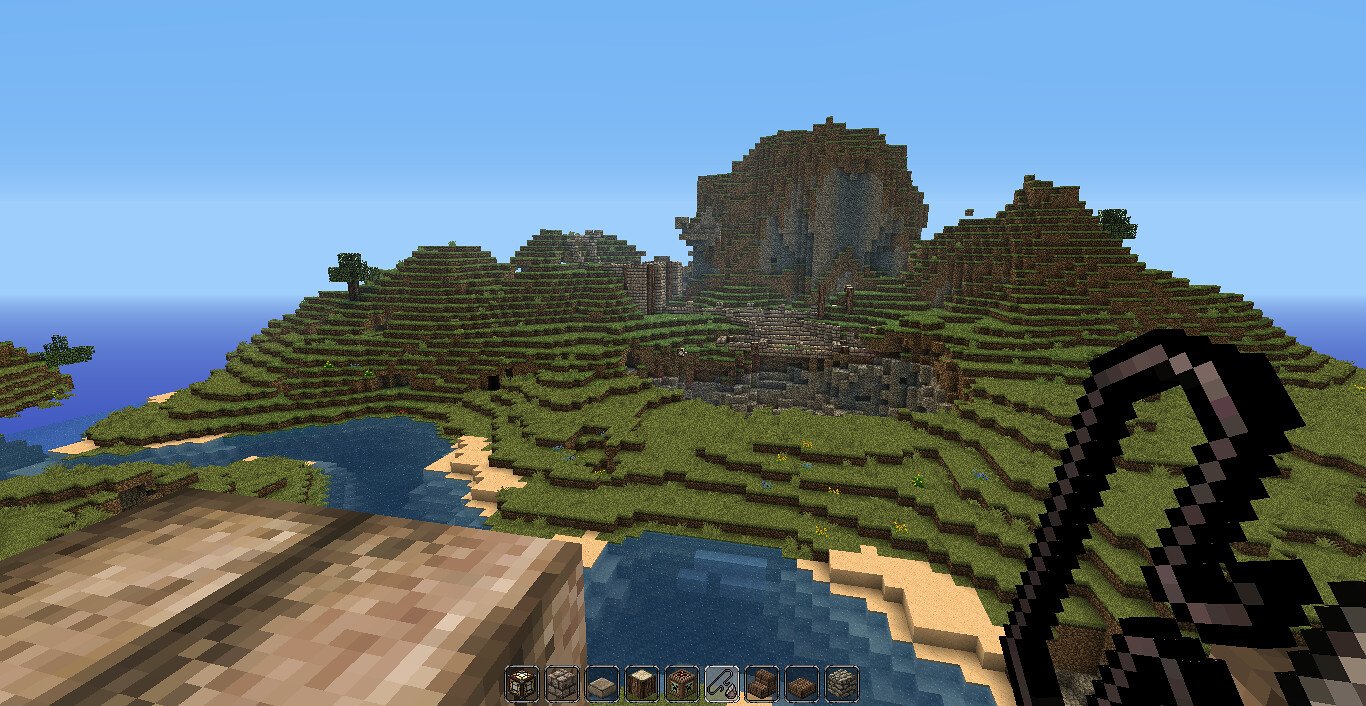This pixelated image appears to be a screenshot from an early video game, possibly from an Atari or ColecoVision console. The scene is depicted in a first-person view, reminiscent of classic games like Doom. The sky is a lighter blue, contrasting with the dark blue water, creating a serene backdrop. Green grass dominates the lower portion of the image, transitioning into brown pixelated areas that resemble a beach where the grass meets the water. In the distance, indistinct pixel formations could represent either mountains or a castle, adding an element of mystery. In the foreground, a round object is visible, which could be interpreted as a weapon, further emphasizing the first-person perspective. The overall pixelated aesthetic harks back to an era when graphics were simple yet evocative.